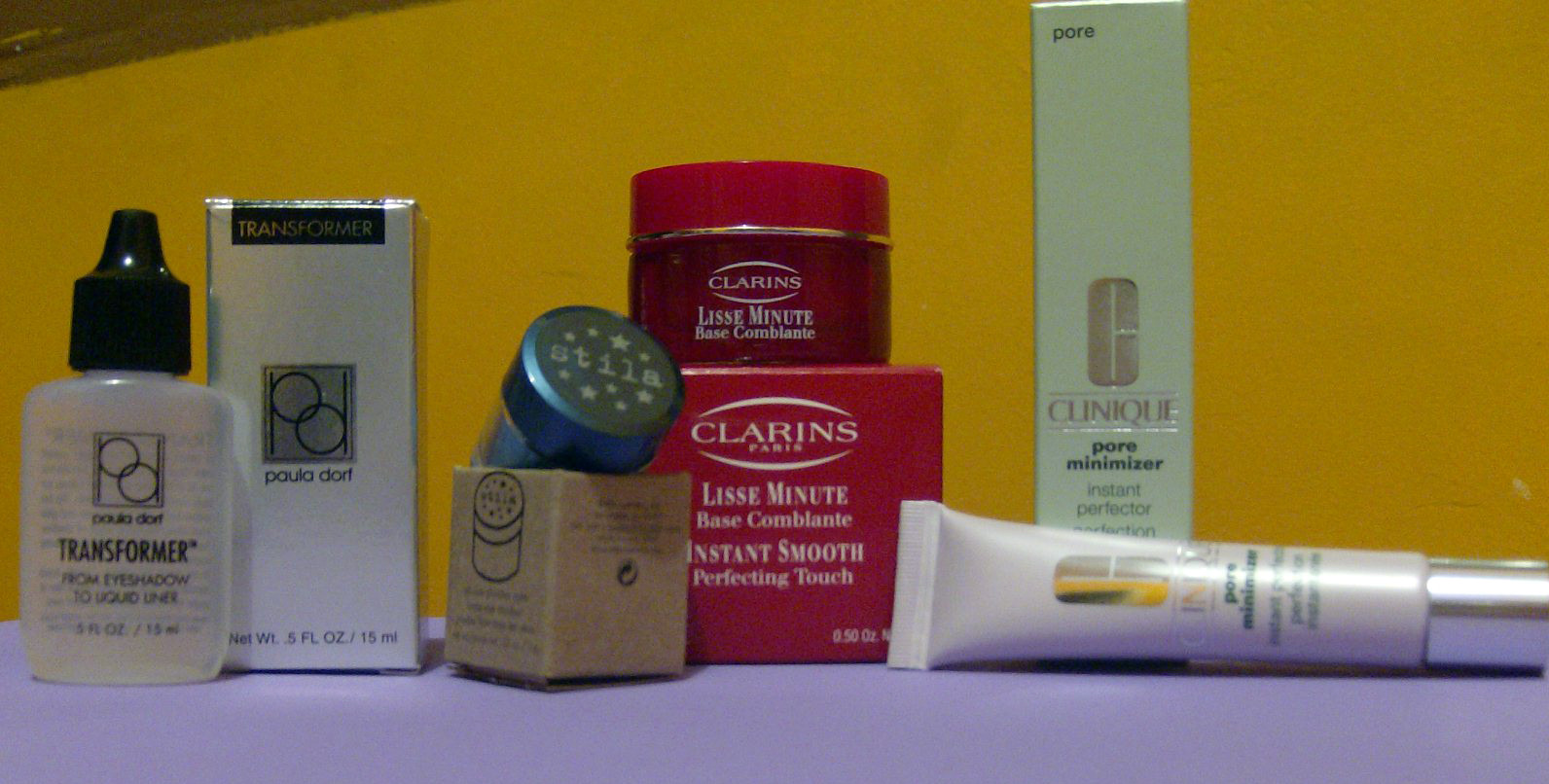The photograph showcases an array of beauty products elegantly arranged on a lavender-colored surface, contrasted by a shimmering gold background. Central to the image is a green Clinique box featuring its logo and a pore minimizer label, with its corresponding tube taken out and placed on its side in front of the box. To its right sits a striking red Clarins box containing a jar of cream, distinguished by its matching red cap. Additionally, there’s another product packaged in a box with a black top, positioned next to the Clarins jar. On the far left, a silver box houses a small bottle filled with clear liquid, capped with a black top. The careful composition and vivid colors of the products create an appealing and luxurious aesthetic.